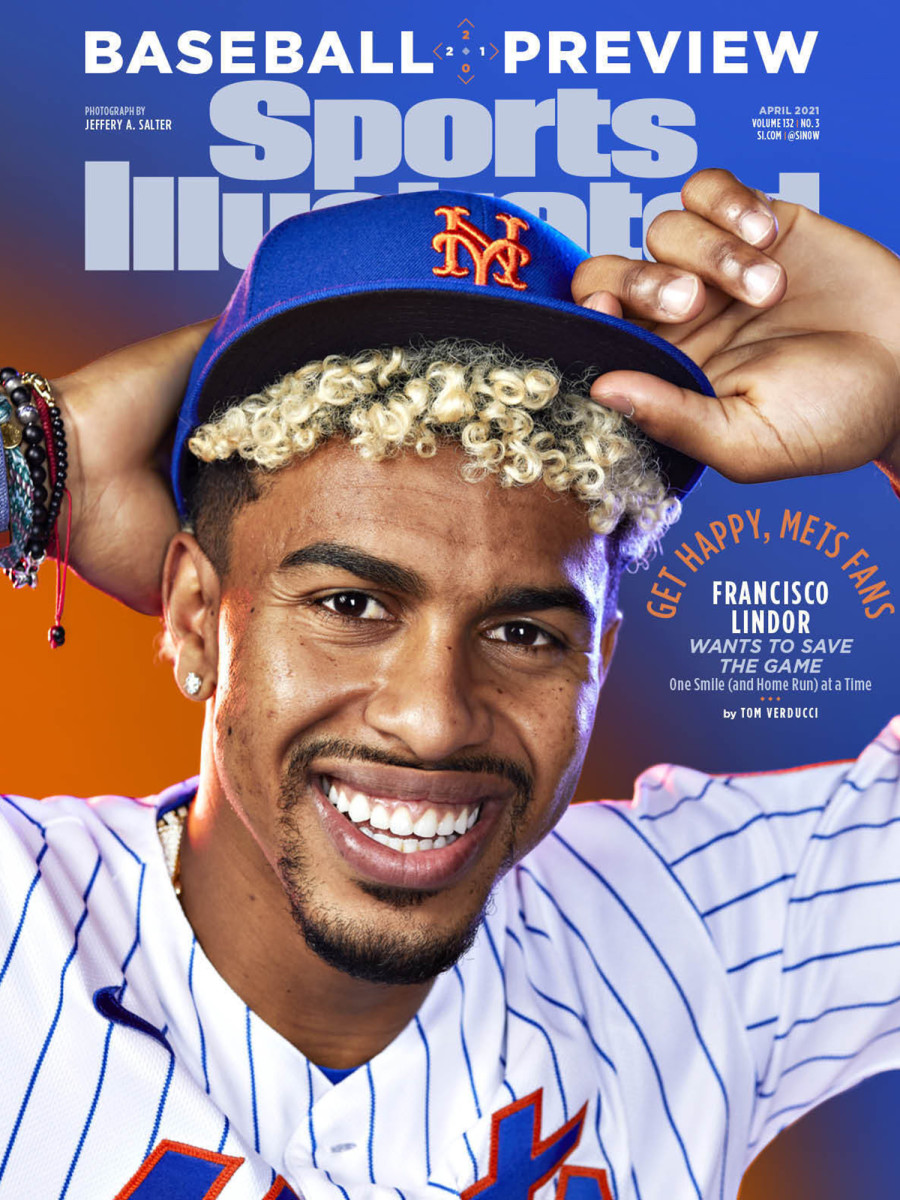The image captures the cover of a Sports Illustrated magazine featuring a Baseball Preview. The prominent figure on the cover is Francisco Lindor, depicted in a Mets uniform complete with blue pinstripes on a white jersey, and a blue cap with an interlocking "NY" logo in orange. The text highlights the cover theme with "Baseball Preview" in white letters at the top, followed by "Sports Illustrated" in grey just below it. A headline to the right of Lindor's smiling face reads, "Get happy, Mets fans, Francisco Lindor wants to save the game one smile and home run at a time," authored by Tom Verducci. The composition includes a tan background interspersed with black, white, blonde, red, light blue, darker blue, and orange colors. The overall setting presents a vibrant and dynamic introduction to the magazine’s baseball season content.